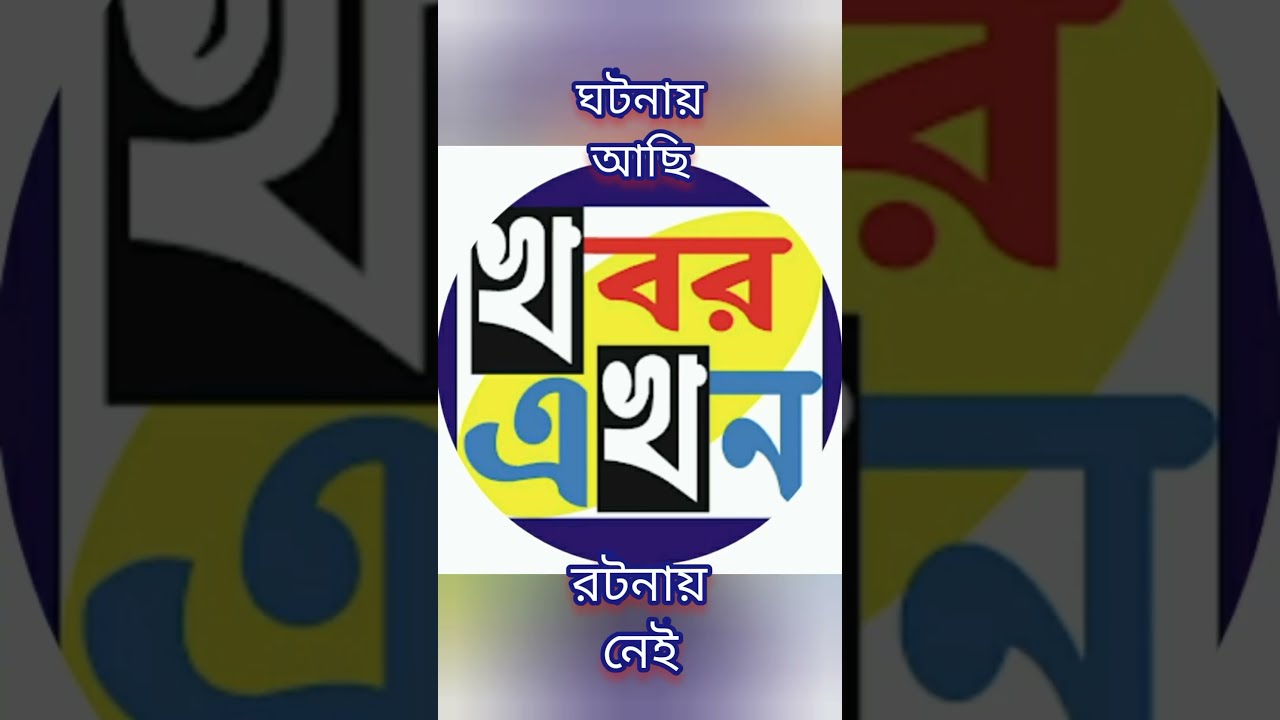The image features a complex design with multiple layers and colors. At the center, there is a vertical, white rectangular image superimposed on a horizontal, light purple background. The central rectangle includes a dark blue-bordered circle set within it, with a yellow oval running diagonally from the lower left to the upper right inside the circle. The circle contains various inscriptions and symbols in red, blue, and white. Above and below the circle are lines of white text with a blue shadow. Outside the central circle, the background features enlarged and muted symbols identical to those inside the circle. Additionally, scattered around the design, there are several black boxes with white text, and numerous blue interspersed letters. Text in white with a blue outline is present both at the top and bottom of the main rectangle, blending into the overall composition. The script appears to be Arabic or a similar language, accompanied by vivid color contrasts and intricate detail.